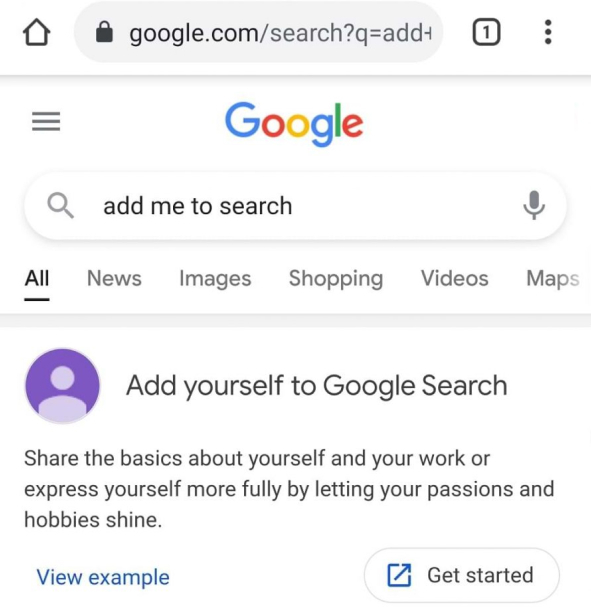## Detailed Caption for a Google Search Page Screenshot:

The image depicts a Google search page within the category of websites. At the top of the page, there is a search bar displaying the URL "google.com/search?q=add...", indicating a search query has been entered. The presence of a lock icon beside the URL confirms that the site is secured. Adjacent to the search bar, a house icon enables users to navigate back to the homepage, while a small "1" next to it signals an alert or notification. To the right, a three-dot menu icon allows access to additional options.

Below this header, the distinctive Google logo is prominently displayed, featuring the familiar color scheme: a blue "G," red "o," yellow "o," blue "g," green "l," and red "e." Beneath the logo, another search bar is visible with the placeholder text "add me to search." This bar is flanked by a magnifying glass icon on the left, signifying the search function, and a microphone icon on the right, enabling voice search.

Further down, a menu bar lists various categories: "All," "News," "Images," "Shopping," "Videos," and "Maps." To the far right of this menu bar, there is a generic profile icon depicting a gray person within a purple circle.

A highlighted section follows, encouraging users to "Add yourself to Google Search." This section invites users to "Share the basics about yourself and your work or express yourself more fully by letting your passions and hobbies shine." Below this call to action, a "View Example" button is highlighted, along with a "Get Started" button to initiate the process.